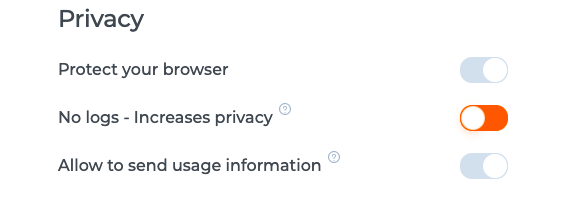A settings interface is displayed on a minimalist white background, devoid of any borders. At the top, the word "Privacy" is spelled out in dark gray text. Below this, there is a section titled "Protect Your Browser" in a lighter gray, with a toggle button next to it set to the "On" position. Further down, a line reads "No logs - Increases privacy," accompanied by an orange "Off" toggle button— a departure from the typical color scheme where 'On' is usually highlighted. The final line states "Allow to send usage information," with a light gray "On" toggle button beside it. At the end of both the second and third lines, a light gray question mark enclosed in a circle icon provides help options. The page is notably free from any other content, emphasizing the stark and clean design.